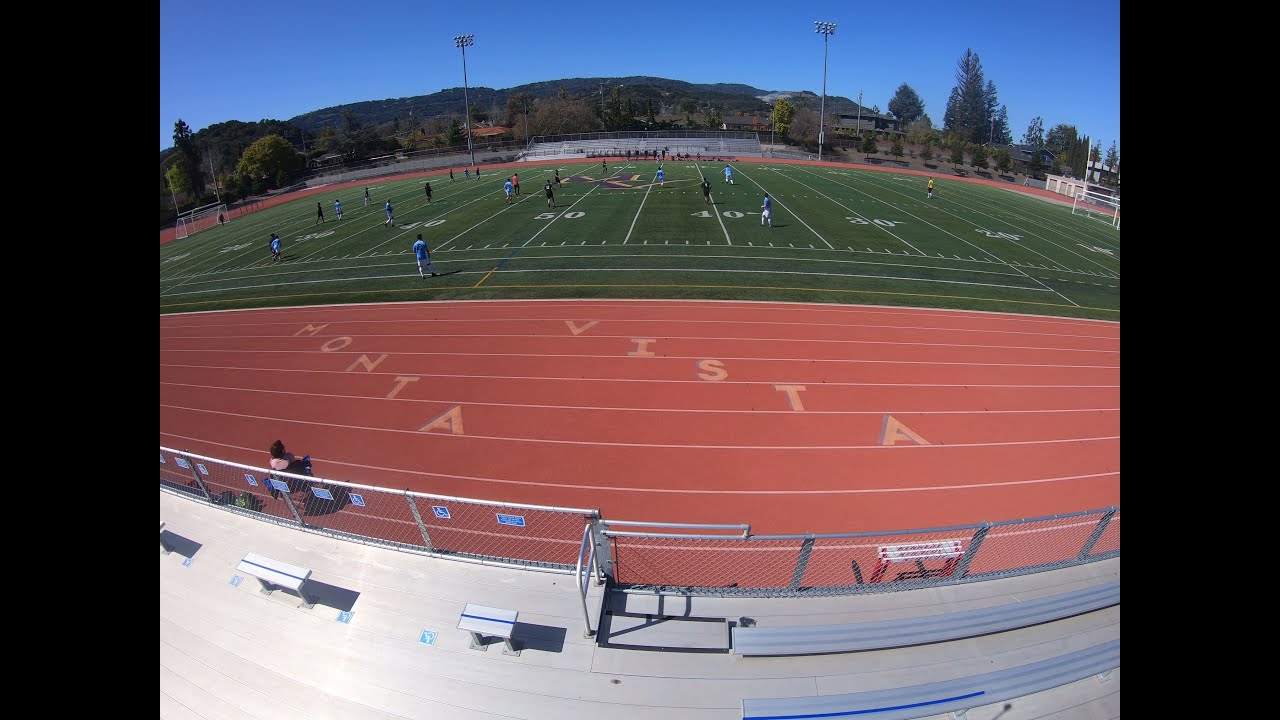The image depicts a high school football stadium named Monta Vista, likely located in California, as suggested by the Spanish name and the mountainous background visible in the distance. The bright, sunny day with clear blue skies highlights the lush green football field, which is surrounded by a distinct red track with white lane markings. The name "Monta Vista" is prominently imprinted on the track. The field is lined up for both football and soccer, with visible goalposts and soccer nets at either end. The stadium is devoid of spectators, indicating that it's a practice session. Numerous players dressed in blue and black uniforms are scattered across the field. The photo appears to be taken from the stands, where you can see the empty bleachers in the foreground and on the opposite side. A single person is seated inside the fence that encloses the football field, positioned on the sideline adjacent to the red track. The surrounding landscape features abundant trees and softly rolling hills, adding to the picturesque setting.